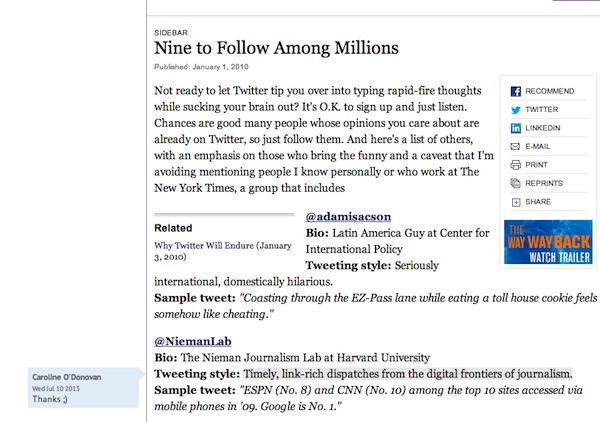In this image, there is a detailed view of an article with the title "Nine to Follow Among Millions" prominently displayed in large font. The article, published on January 1, 2010, includes smaller, gray-colored text just beneath the title indicating the publication date. Below this, a paragraph begins with, “Not ready to let Twitter tip you over into typing rapid-fire thoughts while sucking your brain out.”

Towards the middle of the image, it showcases a Twitter handle, @AdamIsACon, along with a bio and tweet sample. Additionally, at the bottom of the image, another Twitter handle, @NiemanLab, is shown, representing the Nieman Journalism Lab at Harvard University. The article provides details about the bio and tweeting style for @NiemanLab, noting that it differs from the previously mentioned handle. A sample tweet from @NiemanLab is also included.